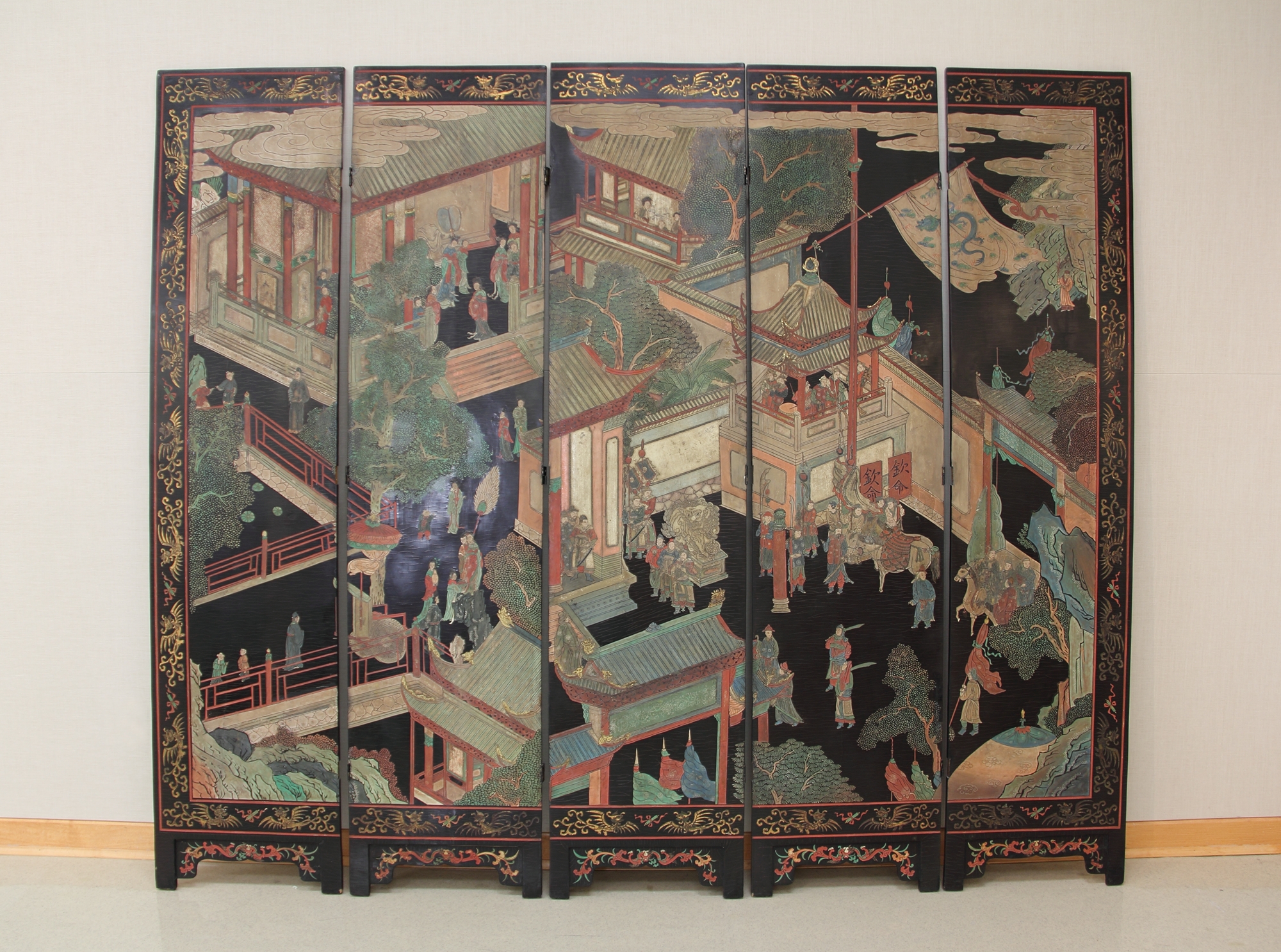This detailed piece of furniture is a five-panel folding screen from the Qing Dynasty, dated around 1676, crafted with lacquer on wood. The screen is painted with an intricate border adorned with gold scrolls, pink and yellow flower vines at the bottom, and gold detailing throughout. The main colors of the artwork are black and gold, with accents of red and green. Depicted on the screen are scenes filled with various elements: men holding samurai swords over their backs, Asian-style houses and huts, and numerous people, some with indistinct faces, who populate the landscape. There's a vibrant sense of life with trees, shrubbery, and horses, including a tan one. In the distance, additional houses and a flag adorned with a blue dragon flutter atop one of the buildings. The floor beneath the screen is shiny linoleum, complementing the light tan baseboard and white wall behind it, adding to the overall ornamental and historical ambiance of the piece.